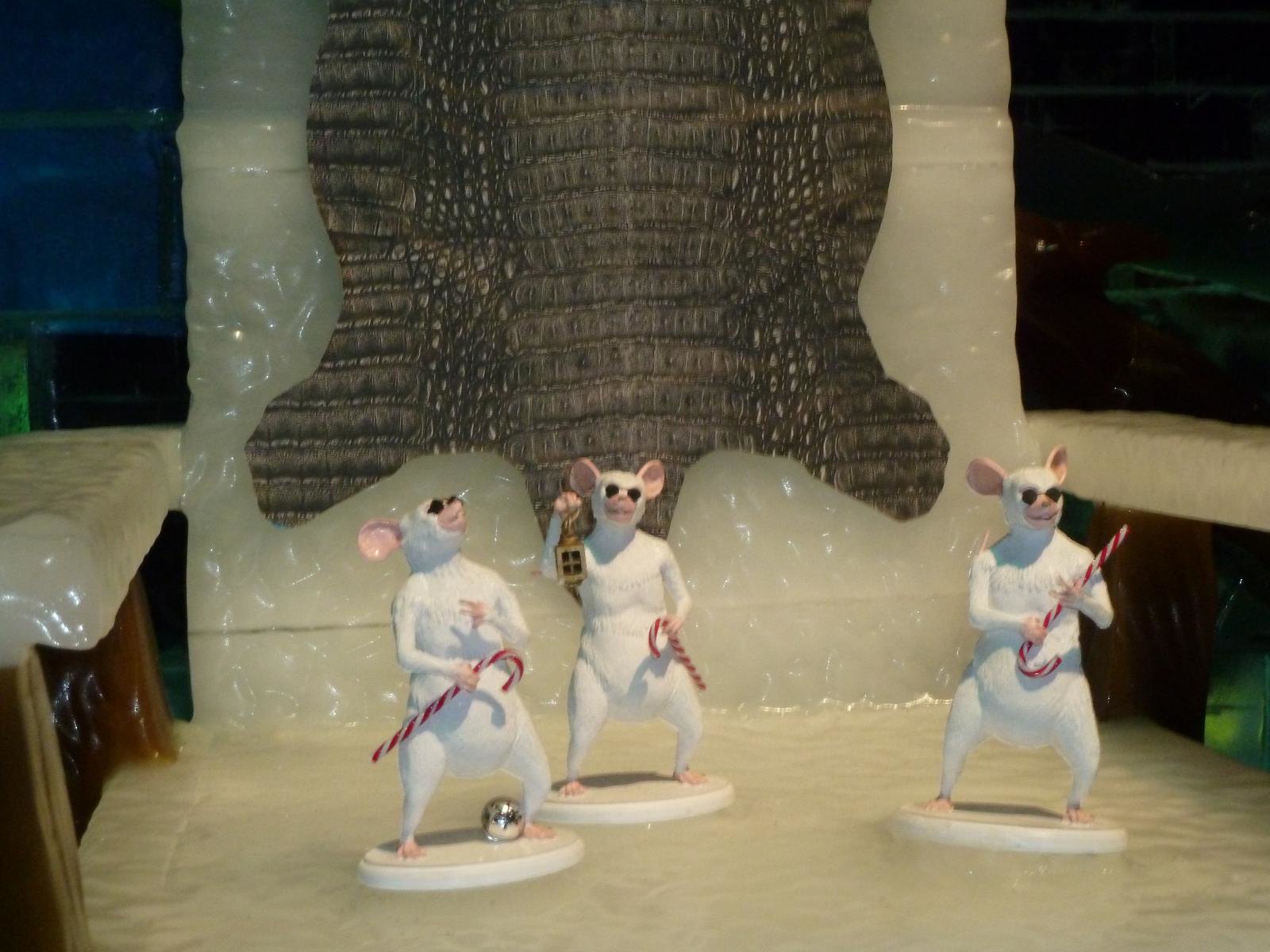The image features a unique decorative artwork showcasing a wooden chair with its arms, back, and seat covered in a substance that resembles beige marble or plastic, giving it an icy appearance. Draped over the back of the chair is a large turtle skin, adding an unexpected natural element to the piece. Positioned on the seat of the chair are three detailed ceramic figurines of mice. Each mouse is painted white with big pink ears and features, and all are wearing dark sunglasses, reminiscent of the "three blind mice" from the nursery rhyme. Each mouse holds a red and white candy cane, suggesting these items serve as their blind sticks. Additionally, one of the mice holds a small golden lantern in its right hand. The figurines are mounted on little oval beige bases, and they are depicted standing upright on their hind legs. The detailed craftsmanship of the mice includes pink accents around their noses and mouths, and the figurine on the far left additionally features a tiny silver ornament on its base, enhancing the whimsical and quirky nature of this eclectic art piece.